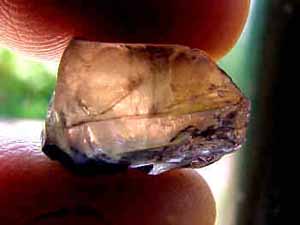In the image, an elderly white man’s dry, visibly aged fingers gently hold a jagged, frosty-looking mineral or crystal in the center of the frame. The rock, possibly quartz or a precious gem, sparkles with a palette of subtle hues including white, blue, tan, and hints of yellow. Surrounding the mineral, the fingerprint ridges on the man’s fingertips are distinctly visible. The blurred, greenish background hints at trees, contributing to a natural, tranquil setting. Sunlight filters through the uncut, jagged edges of the mineral, highlighting its translucent beauty.